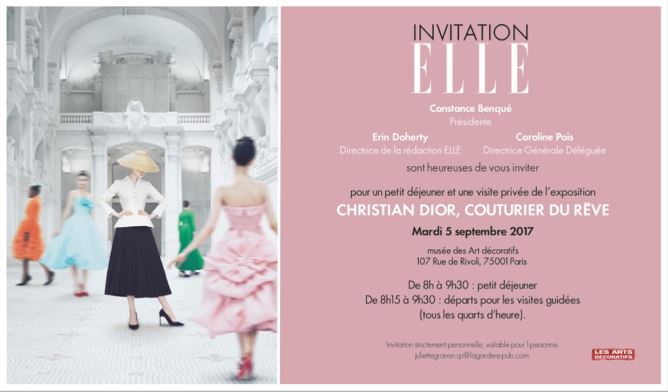The image is a sophisticated invitation card for a private event hosted by the French fashion magazine "Elle." The left side of the card features a striking photograph set in a white marble building, showcasing several models in motion, slightly blurry, wearing elegant dresses. One prominent woman at the center wears a bowl-shaped hat, a black dress, and black high heels. Other models are dressed in a variety of colors, including pink, light blue, green, and orange dresses, each adding to the vivid, dynamic scene.

On the right side of the card, set against a pastel, slightly dark pink background, there is detailed text. At the top, it reads "Invitation" in black font. Below, in a distinctive serif font, is the letter "L", followed by names and titles in sans-serif font: Constance Benkey, Presidente; Erin Doherty, Directrice de la Redaction Elle; and Caroline Poire, Directrice Generale de la Guelle. Additional names mentioned include Alain Saint-Helouz.

Further down, the invitation outlines details of the event: "Pour un petit déjeuner et une visite privée de l'exposition Christian Dior, Comme un couturier du rêve," which translates to "For a breakfast and a private tour of the exhibition Christian Dior, Like a Dream Couturier," scheduled for Tuesday, September 5th, 2017, at the Musée des Arts Décoratifs, 107 Rue de Rivoli, 75001 Paris. Specific times for breakfast and the guided tour are listed as well.

At the bottom left of the invitation, there's a red rectangle with white text that reads "Les Arts," and below runs a black line along the width of the image, adding a refined touch to the overall design.